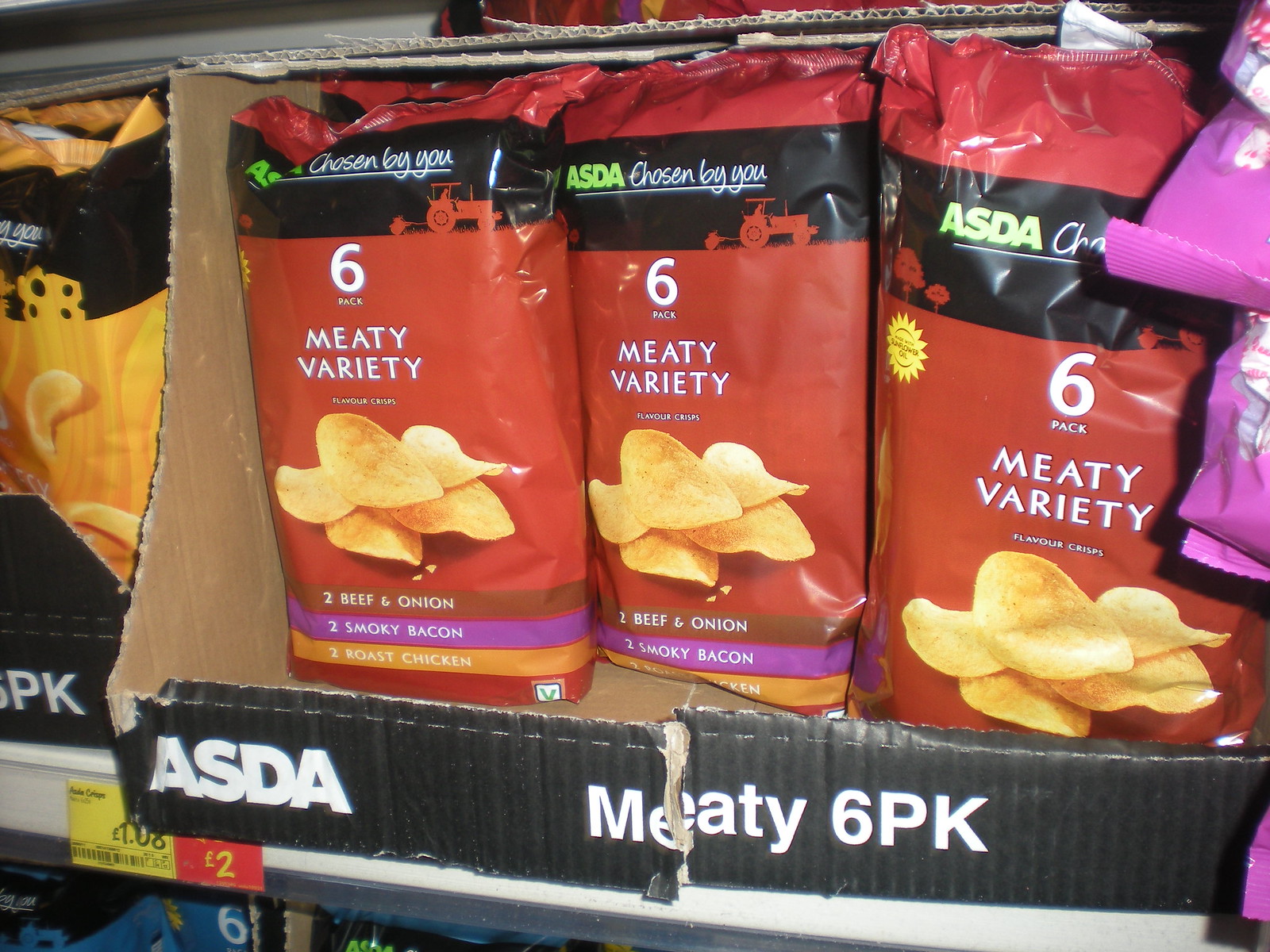This photograph captures a store shelf displaying bags of chips packaged in a partially torn red box with black borders. The box features white text reading "ASDA Meaty 6-Pack," although the torn cardboard disrupts the word "Meaty." Inside the box, there are at least three prominently visible red chip bags, each adorned with a small red tractor on a black stripe. The text on these red bags reads, "ASDA chosen by you," and "6-Pack Meaty Variety Flavored Chips." The flavors specified are "2 Beef and Onion," "2 Smoky Bacon," and "2 Roast Chicken," each flavor differentiated by colored backgrounds—brown, purple, and orange, respectively. The price tag at the bottom corner reads £1.08 and £2.00. The edges of other chip bags are partially visible on the right, but the primary focus remains on the red bags in the center.